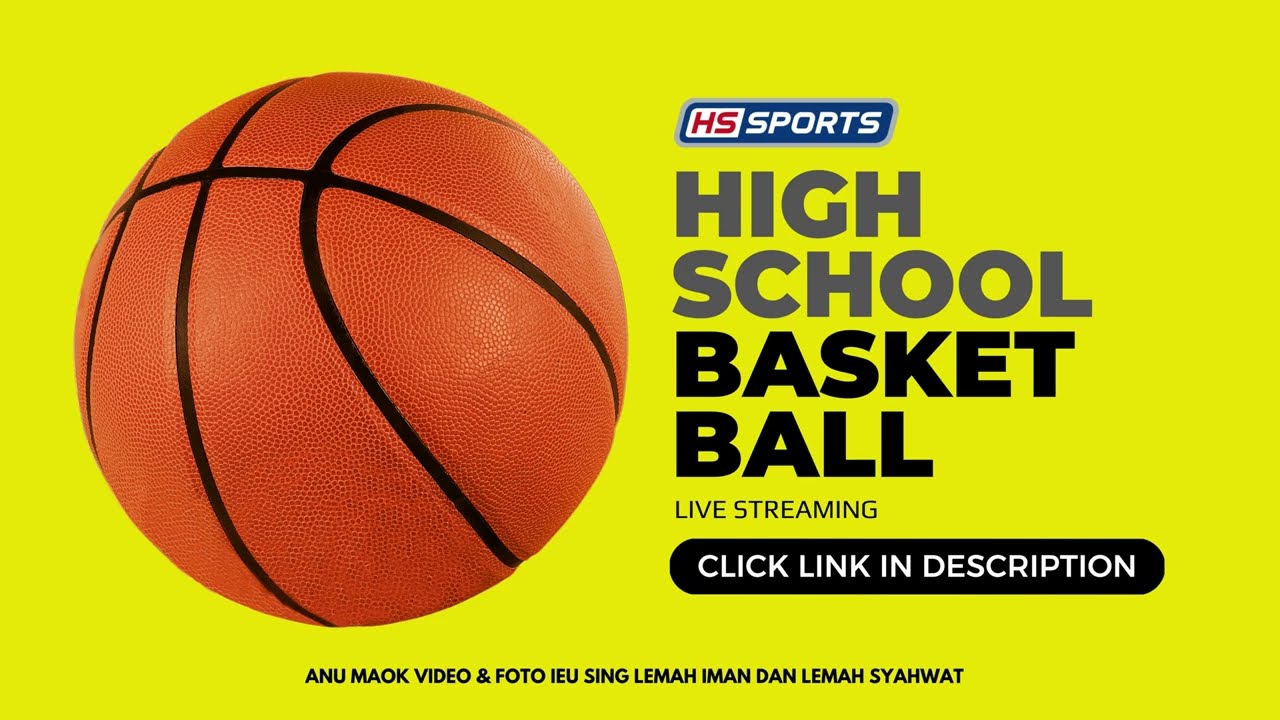The image is an advertisement for high school sports, specifically basketball, featuring a prominent, bright yellow background. On the left side, an orange basketball with black lines occupies a significant portion of the space. Towards the top center-right, there is a small blue box containing a logo with 'HS' in red inside a white background, followed by 'Sports' in white capital letters. Below this, 'HIGH SCHOOL' is written in bold, dark gray capital letters, and directly beneath it, 'BASKETBALL' appears in large black capital letters. Further down, in smaller, narrower text, the words 'LIVE STREAMING' are displayed. Below this section, a black rectangular button contains the text 'CLICK LINK IN DESCRIPTION' in white capital letters. At the very bottom, the text 'A-N-U-M-A-O-K video and photo I-E-U sing L-E-M-A-H-I-M-D-A-N Dan L-E-M-A-S-H-S-Y-A-H-W-A-T' is written in what appears to be a different language, possibly Malay, in black capital letters.